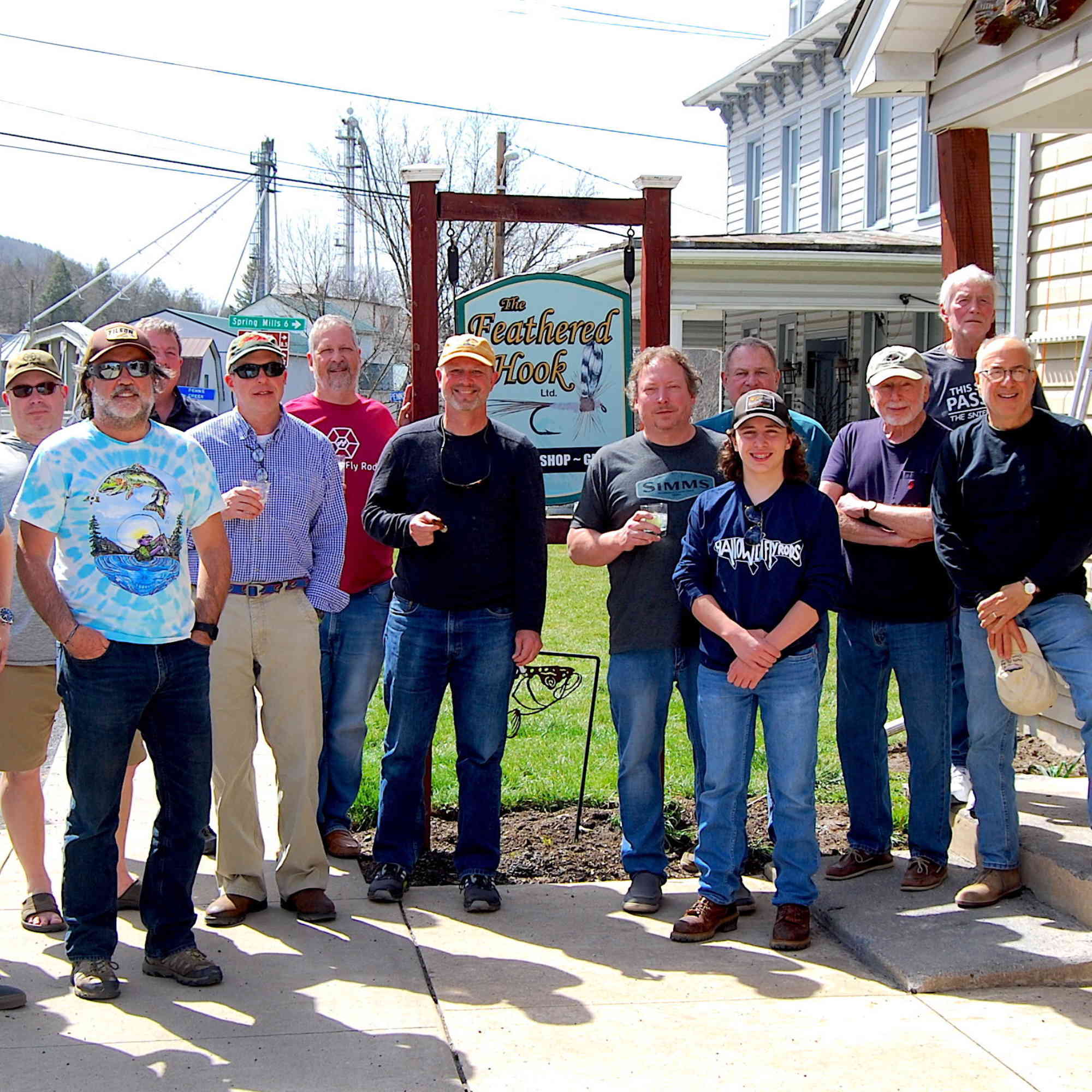In this vibrant digital photograph, a group of twelve predominantly Caucasian individuals, primarily men, and one woman, are casually gathered in front of a quaint establishment called "The Feathered Hook," which appears to be a shop, possibly a tackle or bait shop given the illustration of a fishing hook and lure on the sign. The setting is a sunny day, and the group, most of whom seem to be over 50 years old with gray hair and facial hair, are dressed in comfortable, casual attire including pull-over t-shirts, short and long-sleeved shirts, jeans, and a button-down shirt paired with khakis. Many are sporting ball caps on their heads or holding them in their hands, while two of the men hold glasses containing some sort of drink. The background features a few white houses, lush green lawns, and inviting walkways extending from the pavement where the group stands, all contributing to a friendly, laid-back atmosphere.